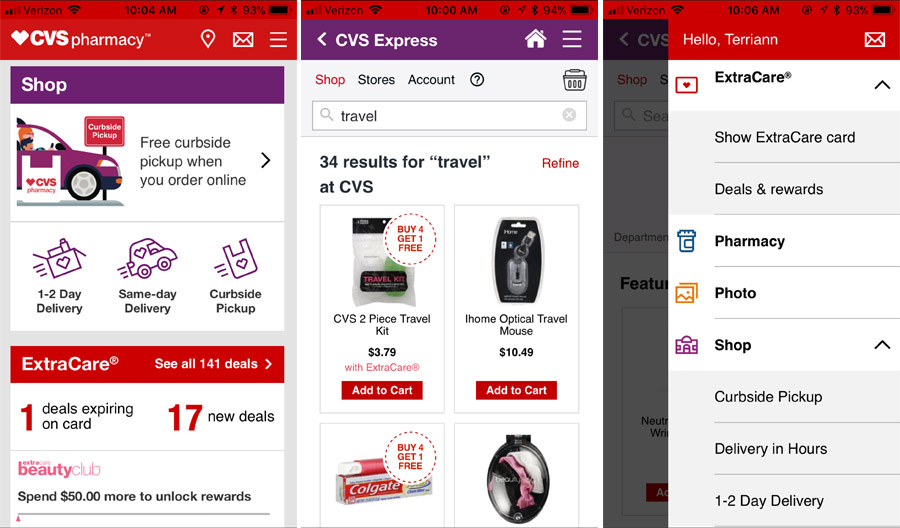This is a series of three screenshots taken from the CVS Pharmacy website on a cell phone. 

The first image captures the top bar showing "Verizon," the time "10:04 AM," and a 93% battery life. Below this, a red banner with white text reads “CVS Pharmacy,” accompanied by a white heart icon next to "CVS." A purple banner labeled "Shop" is visible. The central focus is a cartoon-like illustration of a person driving a car, parked in front of a sign that says "Curbside Pickup." To the right, the text advertises “Free curbside pickup when you order online” with options like “One to two day delivery,” “Same day delivery,” and “Curbside pickup.” Additional information highlights the "Extra Care" program with “See all 141 deals,” including “One deal expiring on card” and “17 new deals” alongside the "Extra Care Beauty Club," which mentions “Spend $50 more to unlock rewards.”

The second image, also taken on a cell phone, shows the time “10:00 AM” and a 94% battery life. The screenshot features the "CVS Express" section with “34 results for travel at CVS.” Prominent items include a “CVS two-piece travel kit, $3.79 with ExtraCare, buy four get one free,” an “iHome optical travel mouse, $10.49,” and a promotion for “Colgate, buy four get one free.” A photograph of a set of hair ties in a black circular case is visible as well.

The final screenshot, taken at “10:06 AM,” features a cell phone bar displaying "Hello Terriam" with “ExtraCare” options like “Show ExtraCare card.” The interface offers navigational links including “Deals and rewards,” “Pharmacy,” “Photo shop,” “Curbside pickup,” “Delivery in hours,” and “One to two day delivery.”